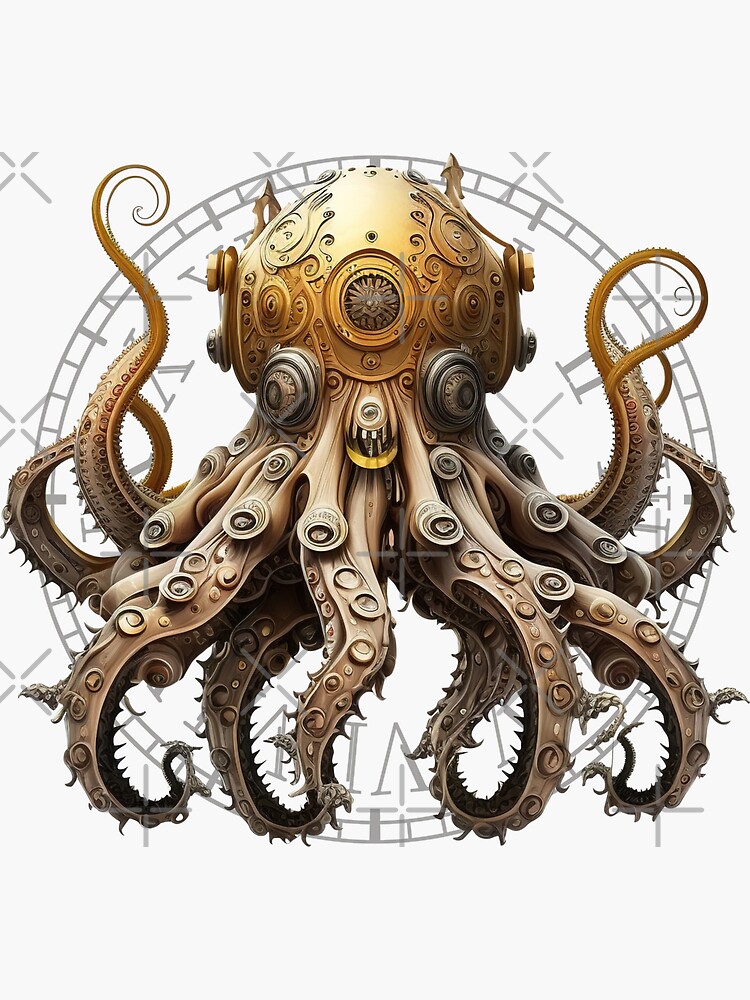This image features a computer-generated artwork of a metallic octopus made from a gold or bronze-colored metal. The elaborate and ornate design is reminiscent of a vintage machine, with its head resembling a decorative diver's helmet featuring swirls, a central round circle, and two circular eyes. The octopus has between eight and ten tentacles, each adorned with circular designs akin to the suckers of a real octopus, and crafted in a two-tone metal: goldish on top and more black underneath. The tentacles grow thinner towards the edges and curl upward. The background showcases a 2D rendering of a clock with Roman numerals in light gold lettering, set against a grey, almost white backdrop. Additionally, small grey crosses are scattered around the clock, further adding to the intricate details of the image.